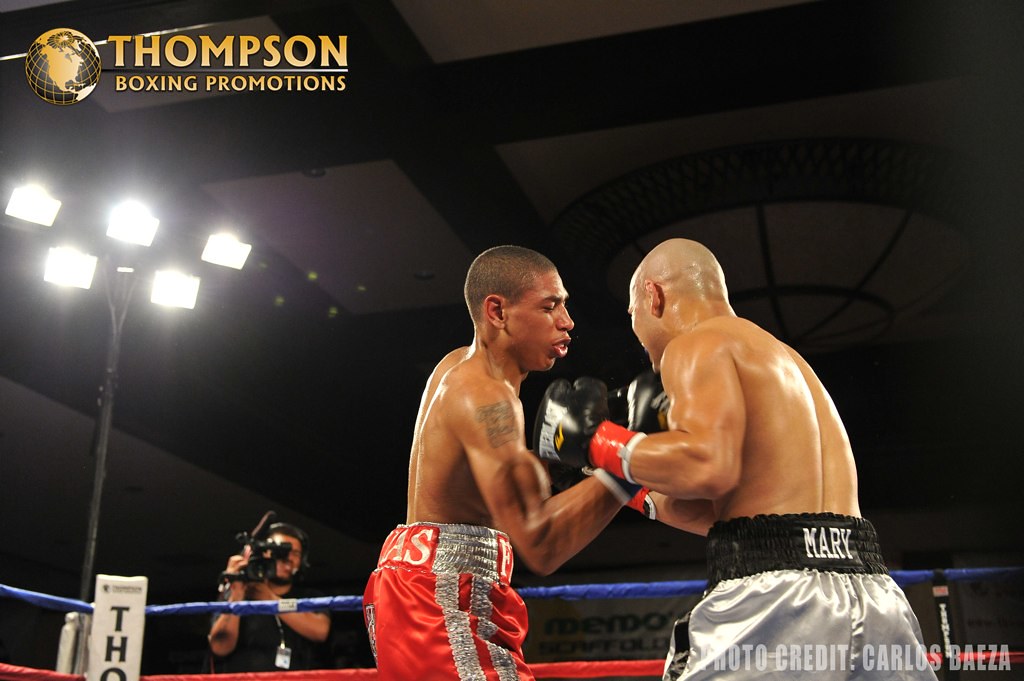This is a detailed, wide-angle photograph capturing the intensity of an indoor boxing match. The image focuses on two shirtless boxers in the ring; the African-American boxer, wearing red trunks with silver Adidas stripes, is delivering an uppercut, while the Caucasian boxer, in silver shorts with a black band that reads "Mary," gears up for a punch. The fighters are close to each other, emphasizing the tension and action of the moment. The boxing ring is visible with its blue and red ropes at the bottom of the image.

In the background, a cameraman with a shoulder-mounted camera records the match, positioned just to the left of a large light fixture with five bright lights illuminating the scene. Positioned prominently, a white post inscribed with the letters "T-H-O" stands just behind the cameraman. Above this scene, the upper left corner of the image displays "Thompson Boxing Promotions" next to a golden globe, highlighting the event's branding. The ceiling of the venue is visible, characterized by large black beams and a curved skylight, suggesting the grandeur of the indoor arena. The bottom right corner credits the photograph to Carlos S-D-A-E-Z-A. The intense, action-packed moment captured against the stark, dark background, with the crowd obscured, focuses all attention on the drama unfolding within the ring.